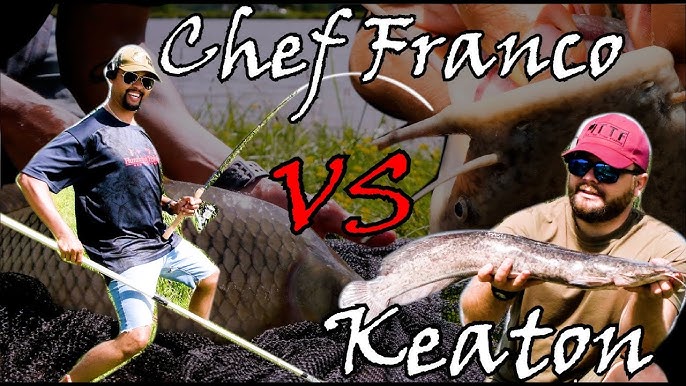The image is a vibrant, eye-catching composition, reminiscent of a YouTube thumbnail designed for clickbait appeal. It depicts a fishing competition between two men: Chef Franco and Keaton. The background is a close-up image showing the arms and hands of two individuals each holding a fish, possibly suggesting a past fishing victory. This background scene includes a visible net, water, and foliage.

In the forefront, prominently photoshopped onto the image, on the left side stands Chef Franco. He is a light-skinned black man, dressed in a black t-shirt with a red graphic, denim cutoff shorts, aviator sunglasses, and a hat. He is holding a bent fishing rod, signaling he has a bite. The text "Chef Franco" in white with a black outline is positioned above him.

On the right side stands Keaton, a white man donning a blue t-shirt, red hat, and sunglasses. He holds up an impressive, long fish that is gray on top and white on the bottom. The text "versus" in red with a black outline sits in the middle, and "Keaton" in white with a black outline is placed at the bottom right.

The overall composition blends action, competition, and a whimsical, possibly staged rivalry between the two men, set against a lush, natural fishing environment.